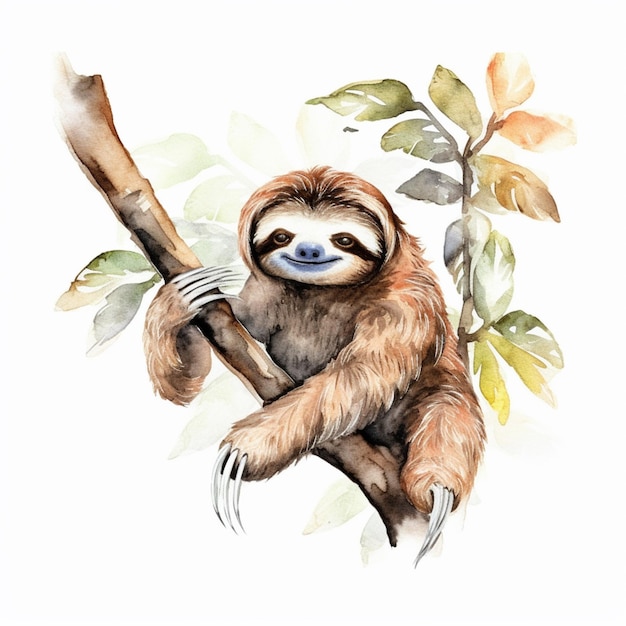This image features a meticulously detailed watercolor painting of a charming sloth perched on a branch. The sloth, rendered primarily in watercolor with some pencil, boasts a rich, textured fur in varying shades of brown—light, dark, and reddish. It has strikingly long, white claws and a face that exudes tranquility and subtle happiness. The sloth gazes directly at the viewer with warm, brown eyes, a deep dark brown mask over both eyes, and a bluish-gray nose and mouth that suggest a gentle smile.

The background showcases leaves in hues of green, orange, and yellow, painted in a more abstract, loose style that contrasts with the detailed brushwork on the sloth. The foliage provides a vibrant yet somewhat impressionistic backdrop, enhancing the sloth's detailed and almost lifelike presence. Despite the looseness of the background, the overall composition beautifully captures the serene habitat of this endearing creature.